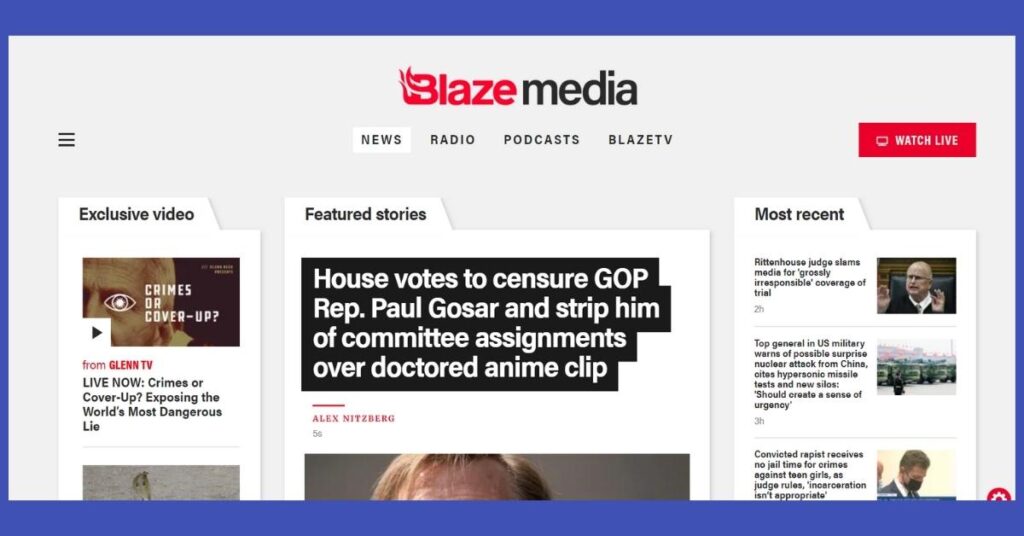A screenshot of the Blaze Media website showcases a well-organized layout with distinguishable visual elements. The page features a refined grayish-white background, framed by a blue outline, offering a clean and structured appearance.

At the top center, the Blaze Media logo prominently stands out. The word "Blaze" is rendered in bold red font with flames extending from the left side of the letter 'B', while "Media" appears in bold black font, highlighting the brand identity distinctly.

Below the logo, four category tabs are aligned horizontally: "News," "Radio," "Podcast," and "Blaze TV." The "News" category is active, indicated by a white box outline, setting it apart from the other tabs, which lack outlines. Additionally, "Watch Live" is displayed in a red box with white lettering on the right side of these categories, while three horizontal lines on the left signify additional menu options.

The content area beneath these categories is divided into three tabs: "Exclusive Video," "Featured Stories," and "Most Recent." Each tab offers specific content tailored to user interests. The "Exclusive Video" tab on the far left provides a selection of exclusive videos. The "Featured Stories" tab in the center highlights notable stories with a distinguished design—a black box heading on a white background—to emphasize its importance. Lastly, the "Most Recent" tab on the right lists the latest articles or videos, ensuring visitors can easily access new content.

This detailed layout and categorization reflect Blaze Media’s commitment to providing an intuitive and engaging user experience.